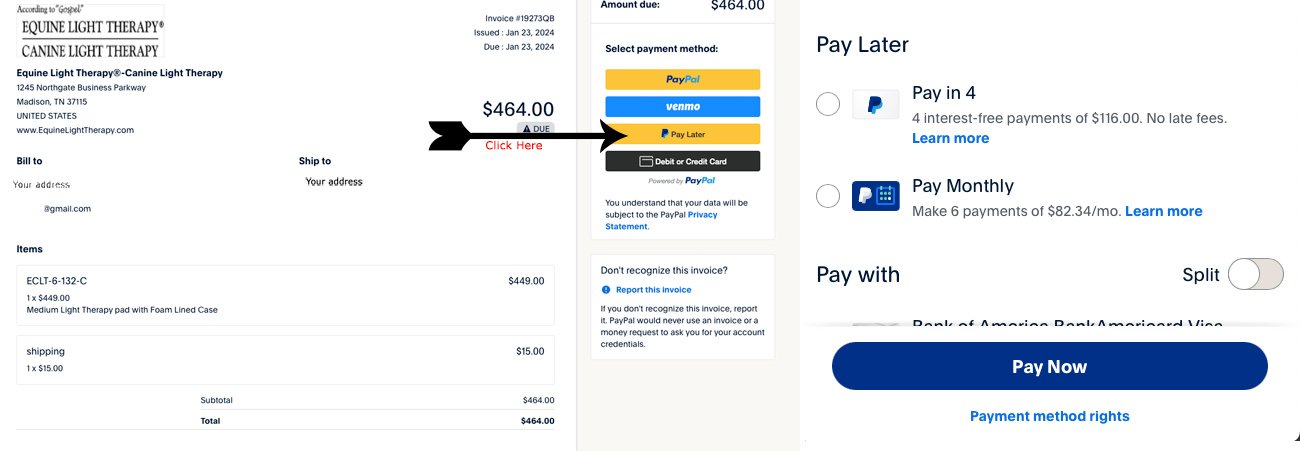Checkout page for an equine and canine therapy store.

The top right corner of the page displays a total cost of $464. A prominent arrow, designed to look like one shot from a bow, points towards a yellow box labeled "Pay Later with PayPal."

The page is divided into three sections. The first section shows an "Amount Due: $464" and prompts the user to "Select Payment Method." Below this, there are options for various payment methods, including a yellow box with the PayPal logo, a blue box with the Venmo logo, and another option to "Pay Later" with the PayPal symbol. Additionally, there's a black box offering the choice to pay with a credit card. Text beneath these options is too small to be legible.

The second section prominently offers a "Pay Later" option with multiple plans. One circular icon with the PayPal logo explains that the user can make four interest-free payments of $116 with no late fees. Another option allows for monthly payments, making six payments ranging from $80 to $134. There's a "Learn More" link beneath each option.

The third section contains a "Pay with" slider that seems to allow for splitting payments. The section is concluded with a blue "Pay Now" button.